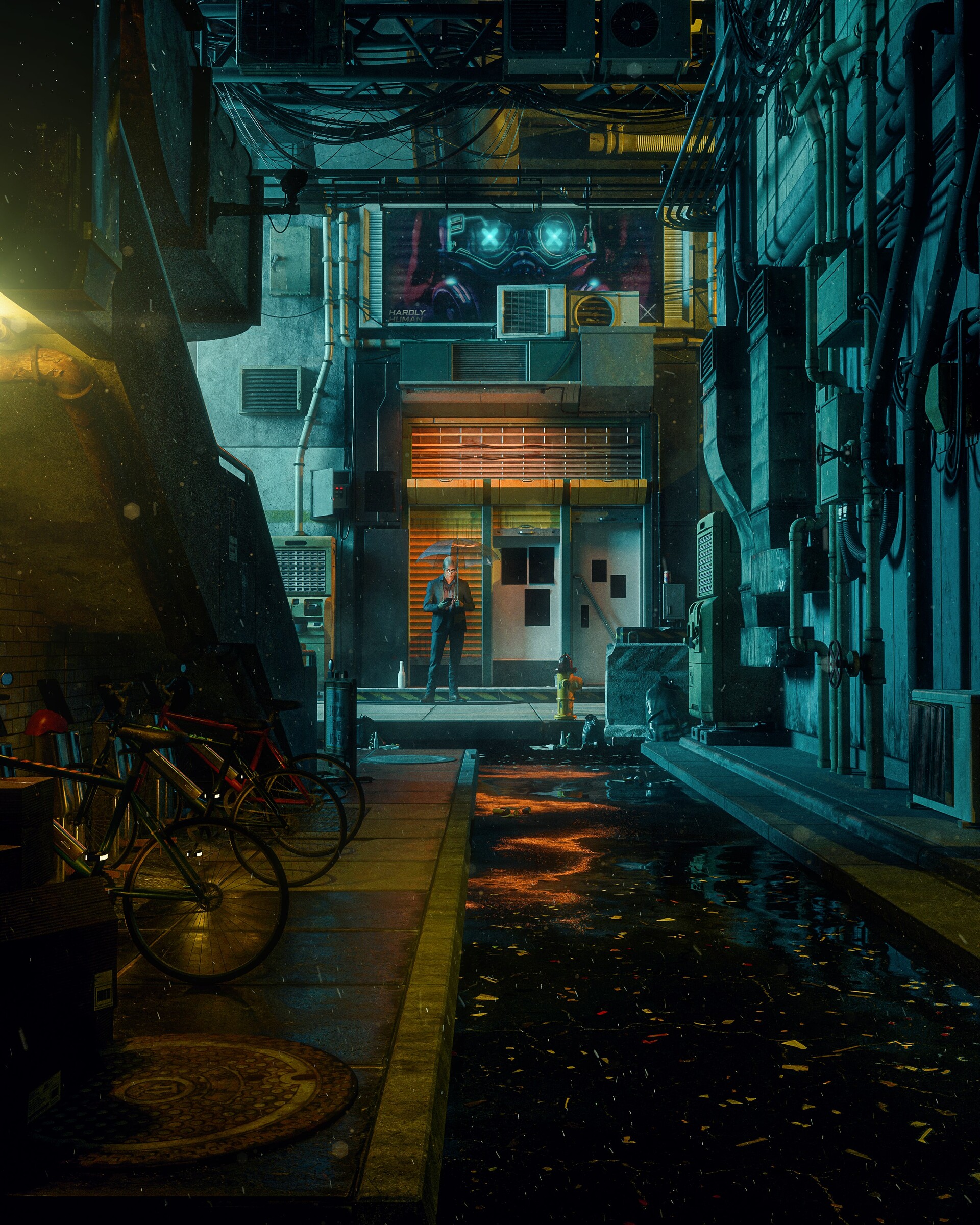The image is a highly detailed, computer-generated piece set in a borderline cyberpunk world, featuring a dark and ominous alleyway. The scene is dominated by a sidewalk littered with bicycles and a manhole cover, to the left side. Adjacent to the sidewalk is a dark, water-filled canal or road with debris floating in it, adding to the dystopian feel. Power lines, electrical equipment, and exposed wires are prominently seen throughout, especially on the right side where a wall is densely packed with conduits and vents.

On the left, there is a staircase with exposed wiring, climbing upwards out of sight. At the far end of the alley, directly in line with the viewer's gaze, stands a man under a dim light, holding an umbrella and a cell phone, possibly near a doorway. Midway down the alley, on the right, another figure appears to be engaged with some kind of device, perhaps a clipboard.

The most striking element of the image is a giant robotic figure hovering above the man with the umbrella. This robot has neon blue X’s for eyes, which stare out from the dimly lit surroundings, creating a focal point of eerie, glowing intensity. While partially obscured, a small, unreadable text or advertisement can be seen near the robot, further adding to the mystery and technological atmosphere of the scene.